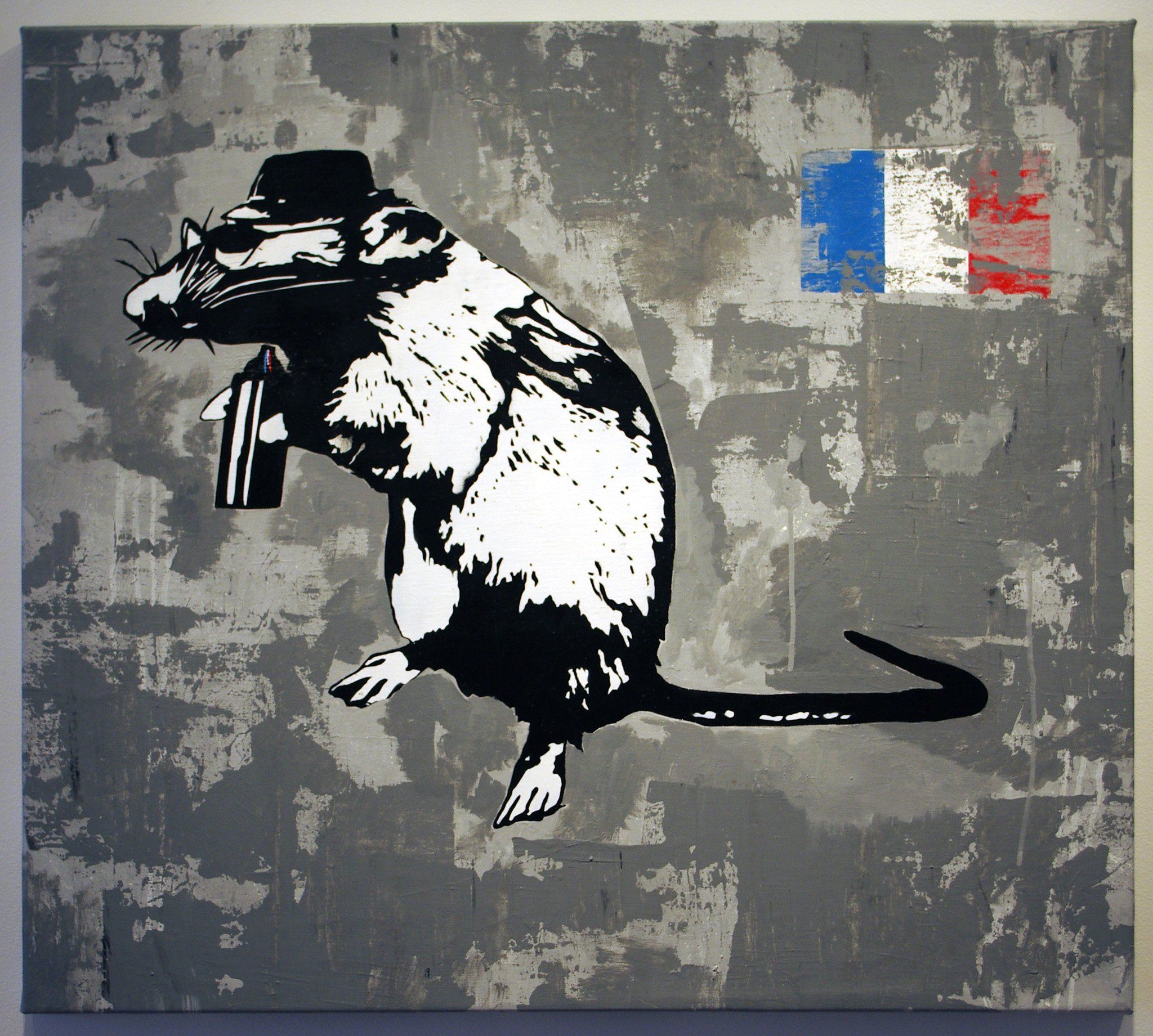The image depicts a large, black-and-white rat standing upright on its hind legs, occupying almost the entire frame. The rat is wearing a vintage hat reminiscent of the 1920s style and a pair of sunglasses that obscure its eyes. It is grasping a flask or possibly a spray paint can in its front paws, which features white reflective stripes and a nozzle, indicating it could be a canister of some sort. The rat’s whiskers are prominently visible, jutting out from its face, and its tail extends into the background.

The background of the image consists of a textured canvas with alternating dark gray, light gray, and brownish paint splashes. In the top right corner, partially obscured by these textures, is a flag in red, white, and blue vertical stripes, which appears to be the French flag. The painting has a light gray border framing the main subject, enhancing the contrast of the central black-and-white rat against the muted, multicolored backdrop.